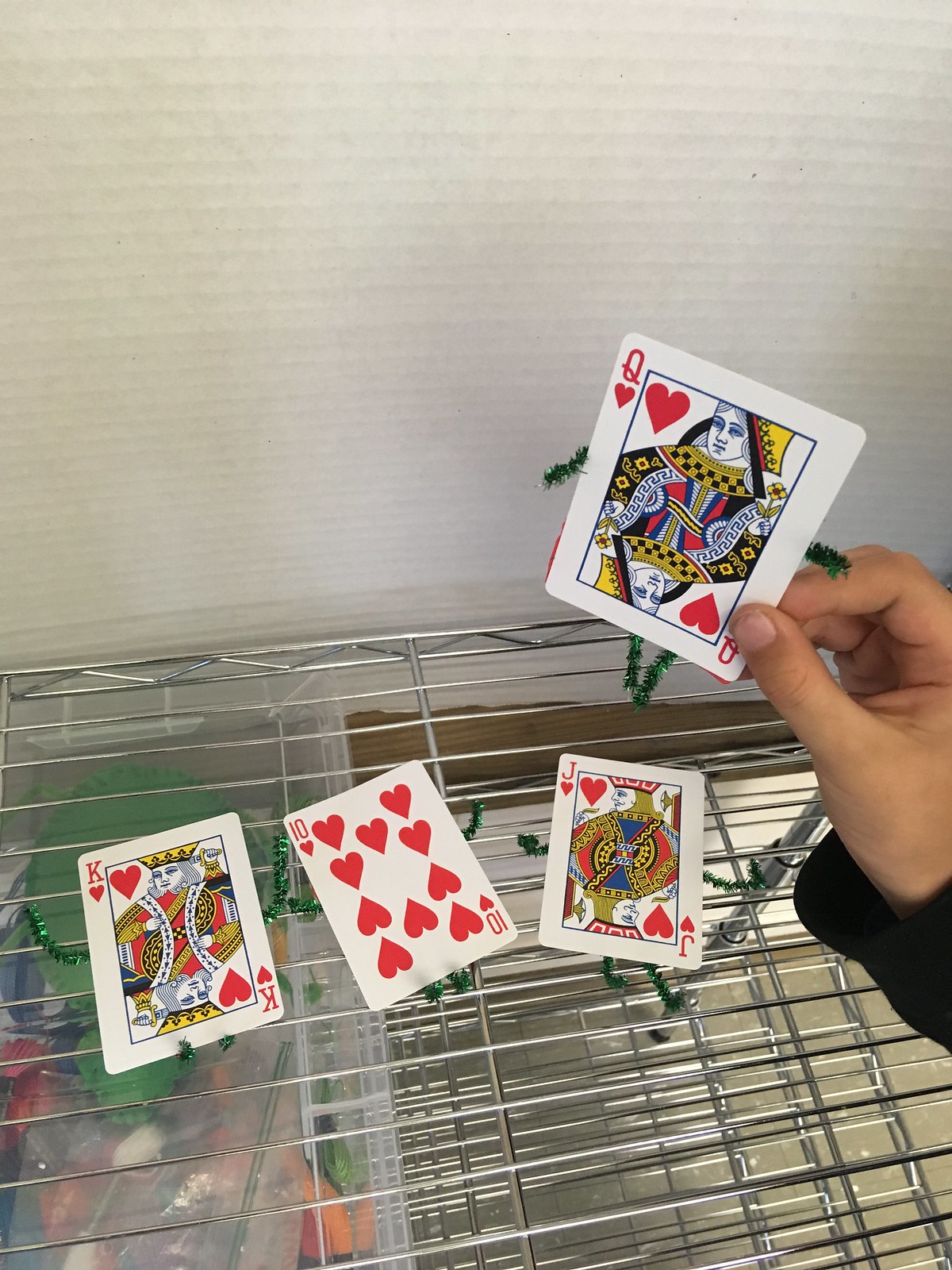In this image, a hand wearing a black sleeve is holding up four playing cards against a white wall with gray horizontal lines resembling notebook paper. The foremost card, held delicately between the person's fingers, is the Queen of Hearts. This card features a white background with a 'Q' and a heart symbol on the left side, enclosed in a blue square, depicting the queen both right-side-up and upside-down, with the 'Q' and heart symbol mirrored. 

Below the Queen of Hearts, three other cards are visible. The Jack of Hearts is placed further down, followed by the Ten of Hearts, and to the far left, the King of Hearts. These three cards rest on what appears to be silver metal racks, layered in multiple levels. Beneath the King of Hearts, an area with plastic and a green material, potentially fabric or another substance, can be seen, positioned just below the intricate arrangement of silver bars that run horizontally and vertically.